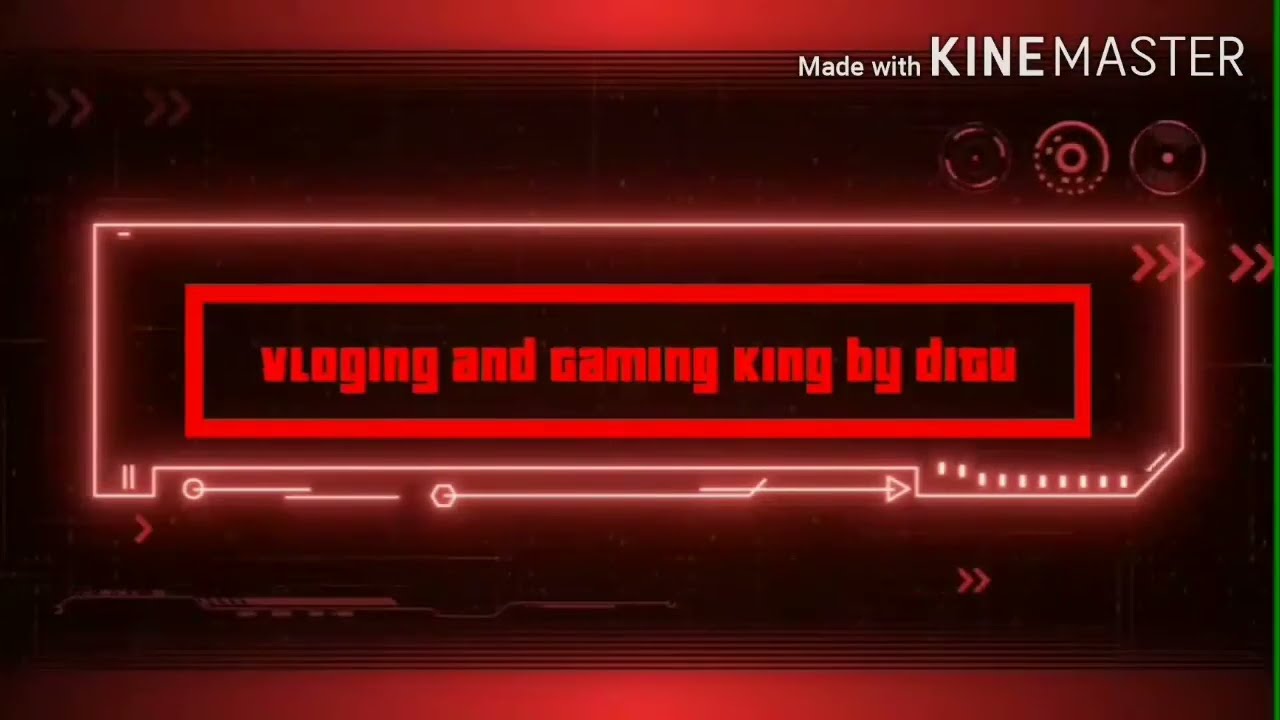The image features a banner with a predominantly dark red background, accented by a black border. At its center, a black rectangular area with a red border displays the text "Vlogging and Gaming King" in red font. The author's name, which is difficult to read, could possibly be "Drew," "Dion," "Daegu," or "DITU". Surrounding this central element is another bright red border, giving the appearance of a glowing frame.

Above the central text, in the upper right corner, the words "Made with KineMaster" are displayed. "Made with" is in a smaller, white font, while "KineMaster" stands out in a larger, bold, white font, with "KINE" being noticeably thicker than "MASTER". 

Scattered across the image are multiple white arrows that resemble fast-forward symbols, particularly placed on the left side, in the middle, and at the bottom. Additionally, there are three small, light red circles with dots in the center, placed above the main text. The image's edges fade into a darker red and black, enhancing the vibrant centerpiece.